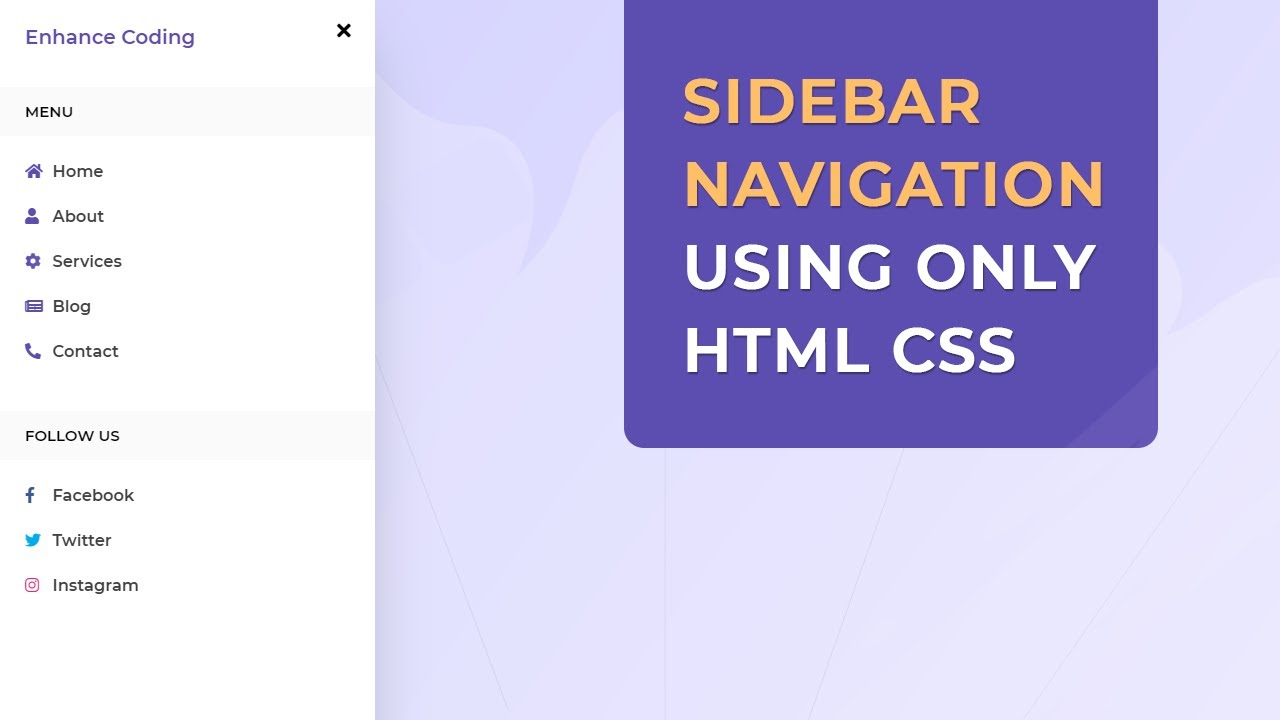In the image, the top left corner prominently displays the text "Enhance Coding" in a vivid purple font. Directly below this, a vertical side menu is positioned on the left side of the image. The menu features various navigational options such as Home, About, Services, Blog, and Contact, each accompanied by a relevant icon. Specifically, the Home option displays a house icon, About shows a person icon, Services has a gear lever icon, Blog features a paper icon, and Contact includes a telephone icon. All these icons are uniformly drawn in purple.

Beneath the navigational options, there is a section labeled "Follow Us," which includes icons for Facebook, Twitter, and Instagram. The Facebook icon is characterized by a blue 'F,' the Twitter icon is represented by a blue Dove, and the Instagram icon is depicted with a purple camera.

On the right side of the image, there is a distinctive box with a purple background that contains another smaller box with a dark purple background. The smaller box highlights text in yellow that reads, "Sidebar Navigation using only HTML, CSS." Notably, within this text, "Sidebar Navigation" is emphasized in an orange font, while "using only HTML, CSS" is written in white. The overall page content appears to be related to Enhance Coding, echoing the title displayed in the top left corner in purple.